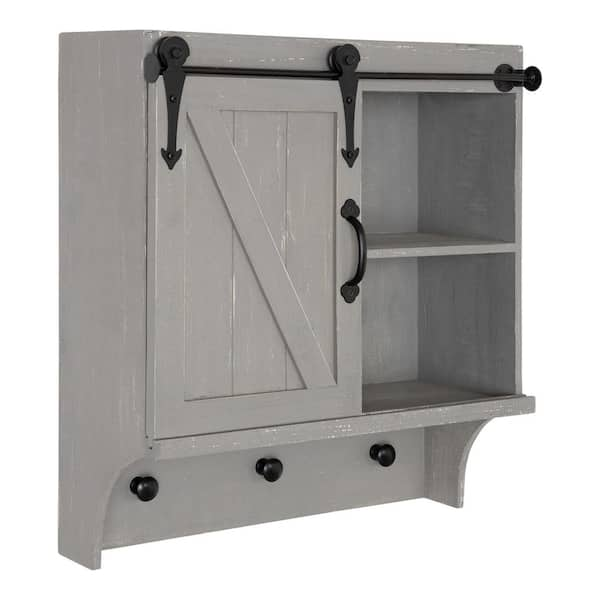The image displays a light gray painted wooden shelf with an integrated cabinet, featuring a barn door design. Photographed against an infinite white background, the shelf is shown from a diagonal angle, allowing a glimpse of a side view. The cabinet door is positioned on the left front side, adorned with a black vertical metal handle and a decorative diagonal wooden slat that intersects three vertical rectangular wood panels, all exhibiting faint white streaks. To the right of the cabinet door, two empty shelves are stacked above each other. Above the cabinet door, there are black brackets and a horizontal black rod. Beneath the shelf are three black metal knobs or pegs, suitable for hanging items such as hats, jackets, gloves, or towels. This versatile piece could be used in various settings, such as a mudroom or bathroom.